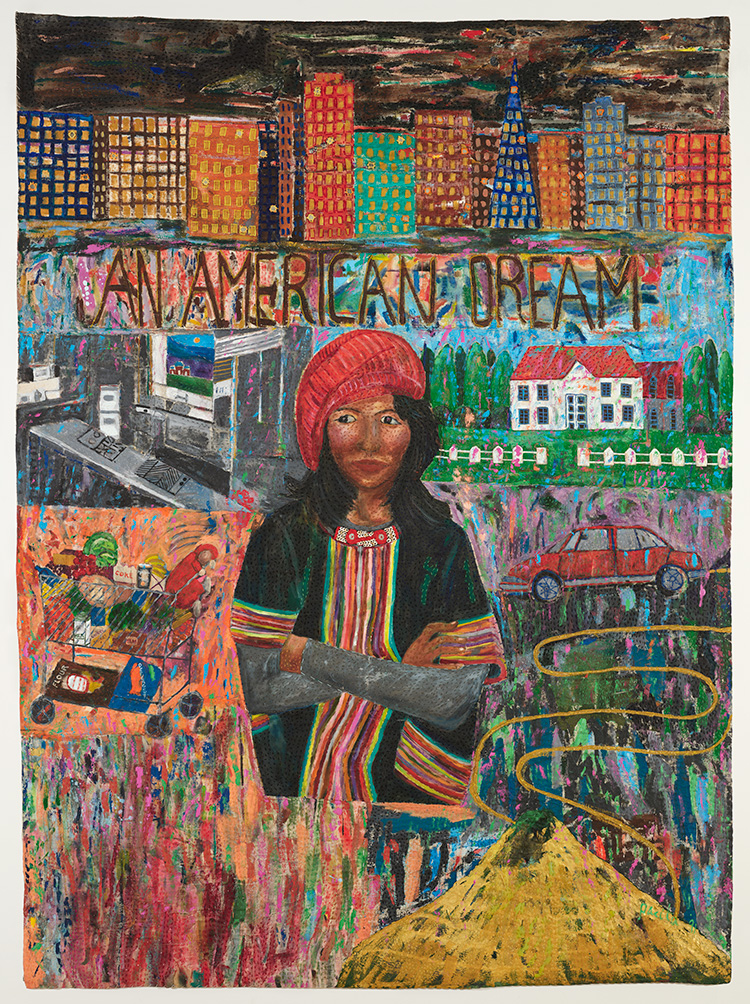This vibrant painting is a blend of abstract and representative art, bursting with color and detail. The top of the painting features a dark sky infused with strokes of blue, green, pink, yellow, and red, setting a complex backdrop. Just below, a row of colorful buildings, varying in shapes from rectangles to triangles, stand tall, each adorned with small yellow windows that resemble city lights. These buildings, painted in hues of blue, orange, red, turquoise, and navy, give an impression of an urban landscape.

Centered prominently is a banner with the phrase "An American Dream" written in black, simple line-drawing letters against a riot of colors, evoking a graffiti wall. Below this banner is a rich tapestry of images: a white two-story house with a red roof and a picket fence stands in one section, while a red car emerges from another. Nearby, a scene depicts a shopping cart brimming with items, perhaps representing consumerism or daily life.

In the heart of the painting lies the focal point—a solemn African American woman. She wears a red beret and a dark green sweater adorned with colorful embroidery stripes along the sleeves and front. Her shoulder-length black hair frames a neutral expression, and her arms are crossed, implying contemplation or defiance. To one side of her, curvy lines resemble a map, leading the viewer's eye around the composition.

Overall, the entire artwork is a kaleidoscope of reds, greens, blues, and blacks, blending structured cityscapes with fluid, freehand elements, capturing the multifaceted experience of the American Dream.